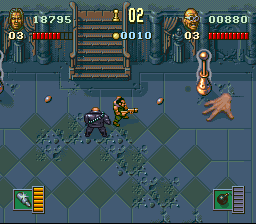This image depicts a screenshot from a video game, showcasing a top-down view of two armed characters standing on a floor adorned with diamond-shaped green and gray tiles. The tile pattern transitions to a more square-like arrangement just above and to the right of the characters. This area is marred with pits, suggesting recent explosive impacts. 

The characters are positioned near each other, forming a 90-degree angle. One figure, a large character clad in a distinctive purple suit and sporting a bullet bandolier, faces the top of the screen. The other character, dressed in a tank top and green pants, faces the right and is in the act of shooting at a large disembodied hand on the floor. This hand is adjacent to a peculiar lamp emitting a strange glow.

The purple-suited character directs his attention toward an imposing stone staircase ascending ahead, flanked by statues nestled in alcoves behind curtains, each supported by pillars. The game's interface at the top displays individual player statistics, including scores, health levels, remaining lives, and various counters. At the bottom, a bomb icon with an empty gauge appears on the right side, while a bullet icon with a full gauge is visible on the left.